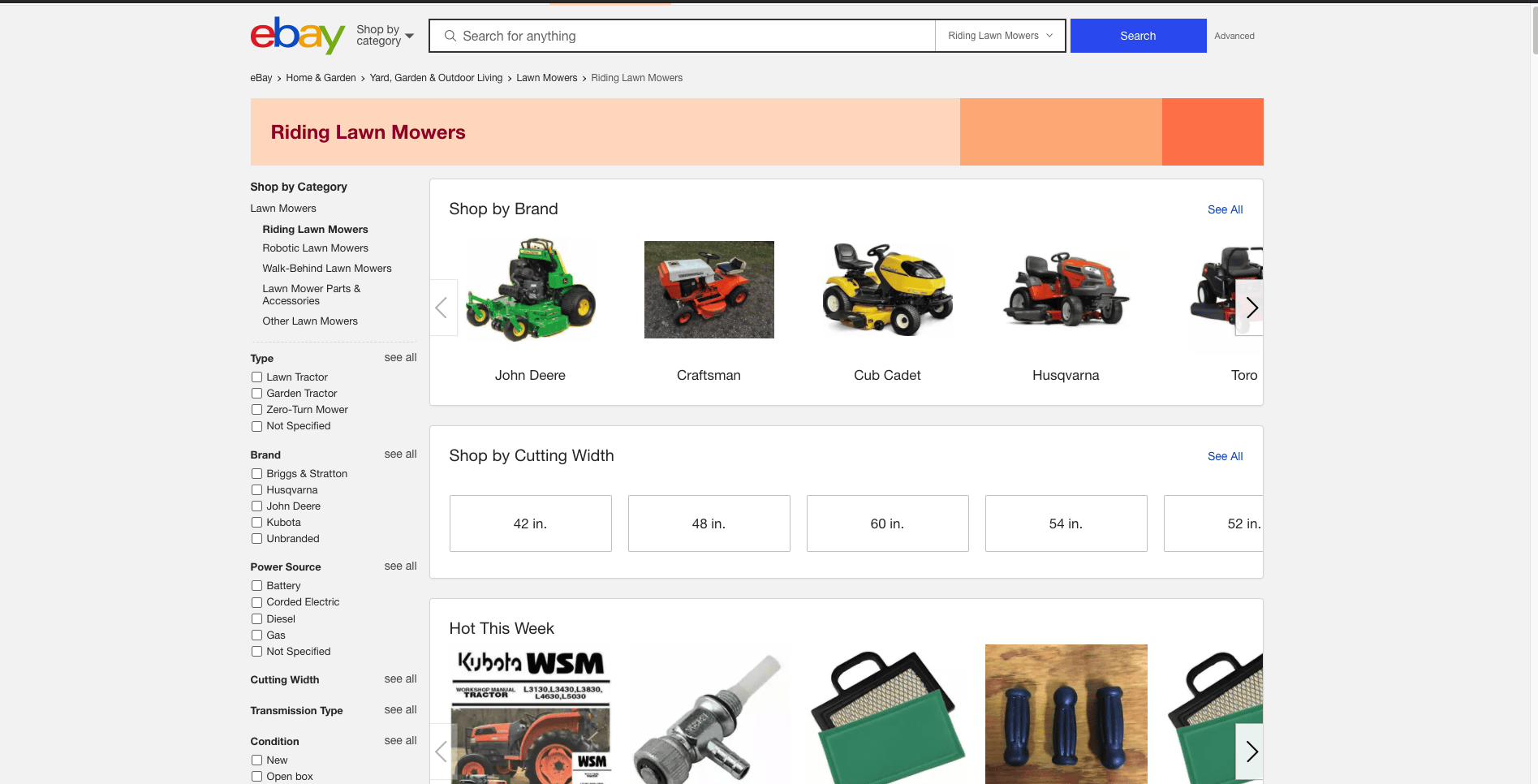This horizontal screenshot captures a webpage from eBay, featuring a pale light gray background. Dominating the page are three white boxes displaying various items. Below the address bar, a light orange and pale pastel orange banner prominently features the red text, "Riding Lawnmowers."

In the top left quadrant, the recognizable eBay logo is displayed, adjacent to a white search bar and a blue search button. On the left side of the page, a vertical column allows users to shop by category, offering filters to select the type, brand, power source, and condition of the desired lawnmower.

The top box, labeled "Shop by Brand," showcases five lawnmowers presented in a horizontal strip. Each mower is color-coded and labeled: green for John Deere, orange for Craftsman, yellow for Club Cadet, red for Husqvarna, and an unlabeled Toro on the far right. The second lawnmower is further highlighted with a gray outline.

Below this section is an area allowing users to shop by cutting width, presenting options through clickable boxes representing different inch measurements. At the bottom of the page, a banner titled "Hot This Week" displays other trending items available on eBay, ensuring users have access to the most popular current products.